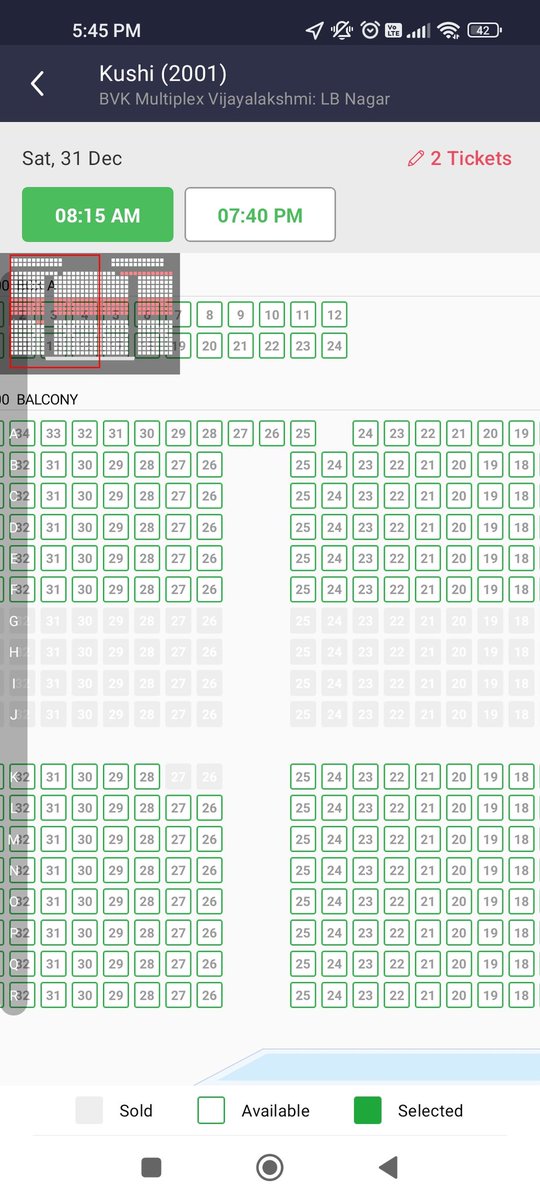This image is a detailed screenshot of a theater or concert hall seat selection interface for an event named "Kushi." The title of the event, "Kushi," is prominently displayed in the top-left corner, accompanied by the year "2001." Below the title, the interface features a grid layout with numerous individually numbered squares, representing different seats across various rows and sections of the venue.

The date of the event is revealed as Saturday, December 31st, with two available showtimes: 8:15 a.m. and 7:40 p.m. In this particular screenshot, two tickets have already been selected. At the bottom of the image, a legend explains the seat selection status: green squares indicate selected seats, while white squares denote available seats.

Additional details are present in the interface. The current time is shown as 5:45 p.m. in the top left-hand corner, and the battery status of the device capturing the screenshot is noted as 42% on the top right-hand corner. The comprehensive display of seat choices and other crucial details gives a clear and organized view for prospective attendees planning to attend the event "Kushi."